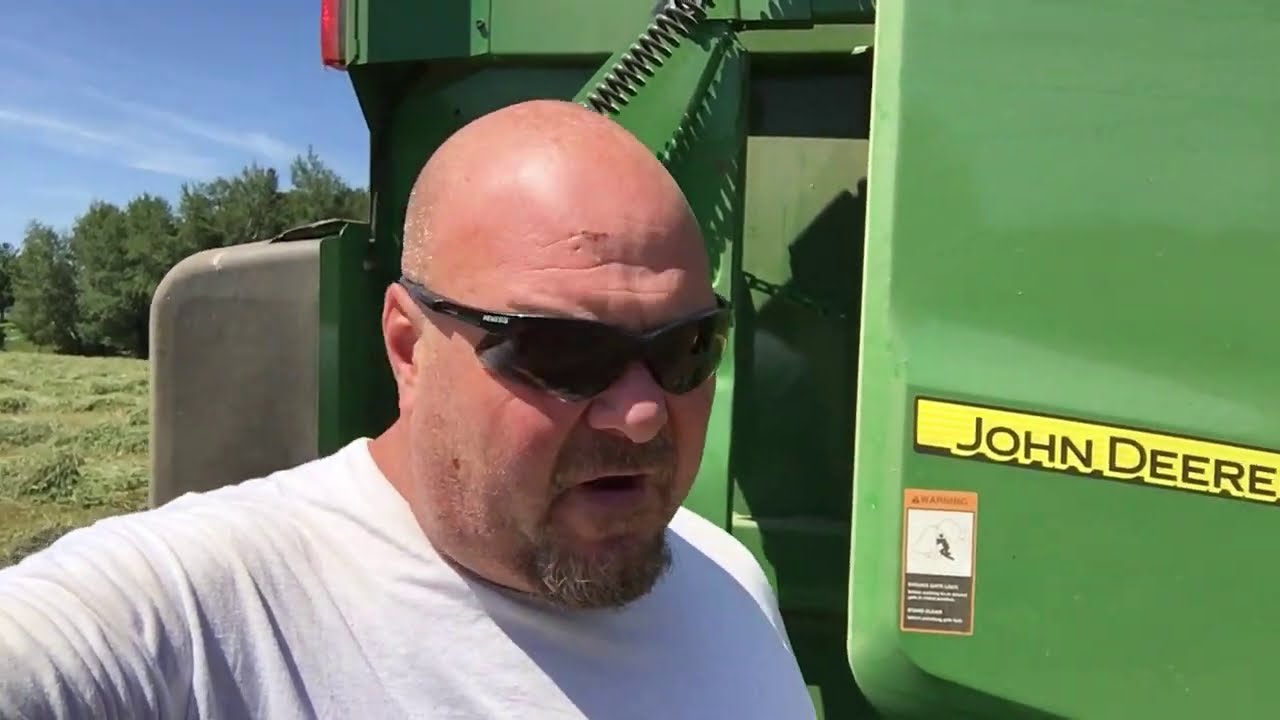In the center of the image stands a bald, bearded man wearing a thin white t-shirt and black sunglasses with dark lenses. He appears to be looking downward slightly to the right, revealing a light-colored mustache and a bit of gray in his beard. Behind him looms a large green tractor branded with the John Deere logo, clearly visible in a yellow rectangle on the vehicle's side. Just below the branding, there's a warning label with an orange frame and a graphic of a person climbing into the vehicle. Over his left shoulder stretches a green field with multiple tall trees in the distance, set against a light blue sky streaked with thin white clouds, indicating it's daytime. The overall scene suggests a quiet, contemplative moment in a rural setting.